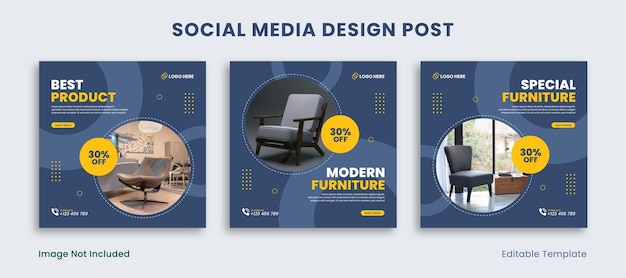The image is an advertisement showcasing a social media design post for furniture with a consistent blue and white theme. The background is primarily navy blue adorned with light blue and yellow circular elements. Three furniture items are featured, each with a prominent "30% off" label in yellow text. The leftmost item is a brown, armless chair with a black metal leg base, tagged as the "best product." In the center, a gray chair is highlighted with a label for "modern furniture," featuring a wooden frame and armrests. The rightmost ad presents a sleek, high-back blue chair, marked under "special furniture." The whole design communicates a clean, modern aesthetic with clear promotional messages, enhancing the impression of a sophisticated social media advertisement. At the top of the ad, the text reads “Social Media Design Post,” and the design is noted to be editable, as indicated by a small label in the corner.